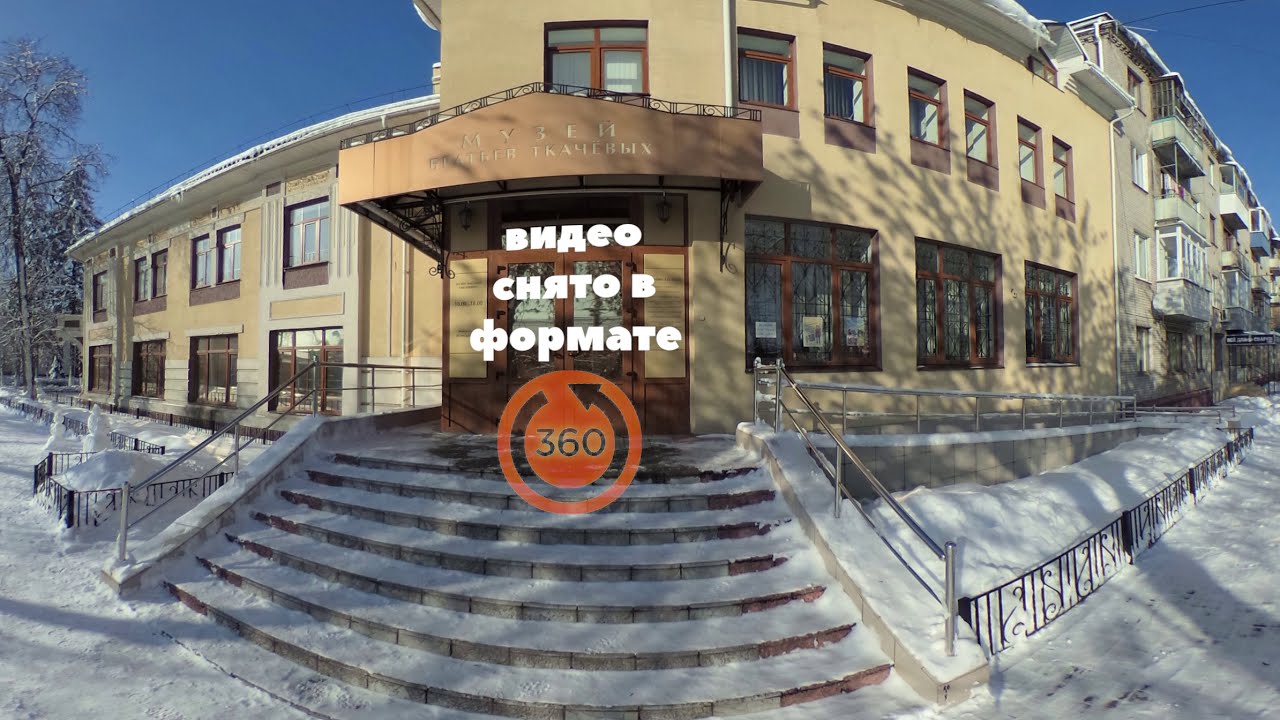In this full-color outdoor photograph taken on a sunny winter's day, we see a panoramic, slightly warped fisheye view of a large beige stucco building with brown-framed windows. The photograph captures the front facade of the building, which consists of a two-story section attached to a three-story segment, creating an overall curved appearance. Snow blankets the ground, the steps leading up to the entrance, and a short black iron fence likely enclosing a garden area now indistinguishable under the snow.

An orange circle featuring a black arrow around its perimeter and the number "360" at its center suggests a 360-degree view aspect of the image. Above the double doors, there is a sign with text in what appears to be an Eastern European language, possibly Russian, though the exact name is unreadable. Silver railings, including a handicap-access ramp, can be seen to the right. To the far left stands a solitary tree outlined against the clear blue sky, adding to the wintery atmosphere of this scene. The building's aesthetic is completed by a large brown awning and a series of neatly arranged, wood-framed windows that punctuate the walls.